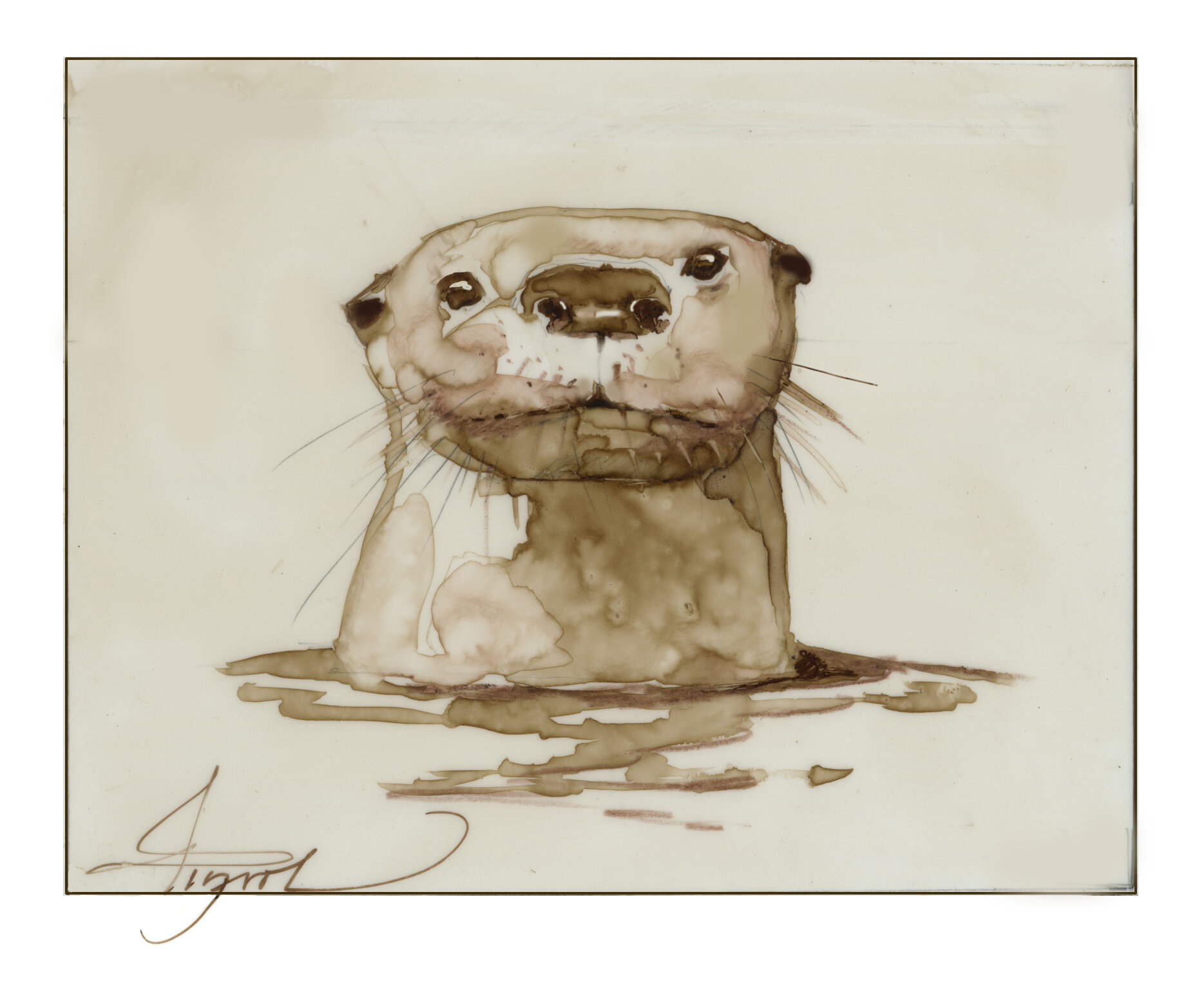This black and white drawing showcases the detailed face of an otter poking its head up out of the water. Set against a white backdrop, the artwork features a black line border that frames the scene. The otter, positioned centrally, has dark, bead-like eyes, a pronounced wide black nose, and tiny ears on the sides of its wide, bean-shaped head. The otter's neck appears thick and round, flaring slightly as it meets the water's surface. Detailed whiskers sprout from its snout, and its mouth is closed. The water's surface is depicted with subtle ripples and darker shades, indicating the disturbance created by the otter's emergence. The overall color palette employs greys and grey-browns, giving it a watercolor-like effect. The bottom left corner of the artwork bears a cursive signature in a loopy, hard-to-read text, providing a unique touch to the piece.